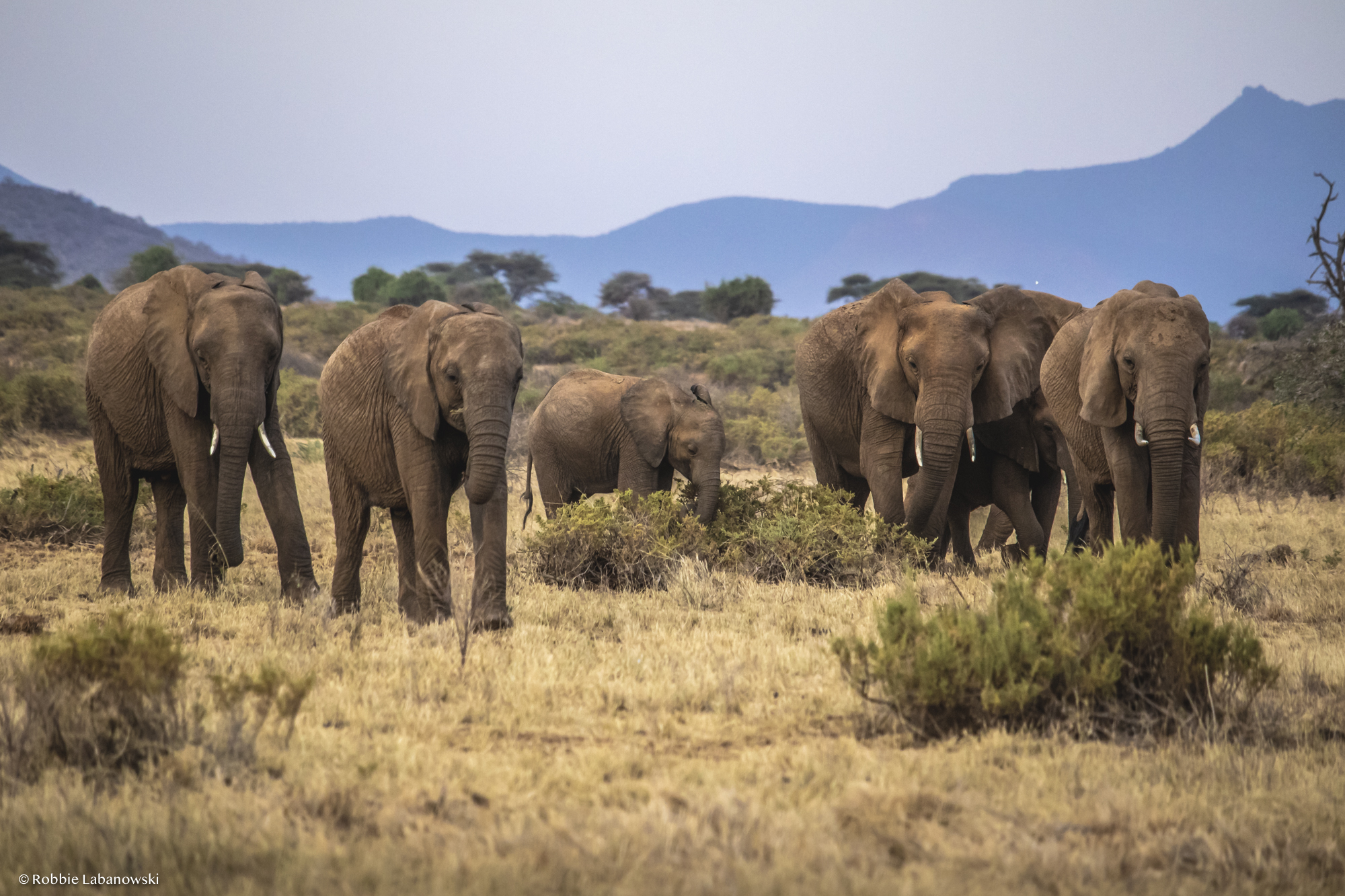A group of six African elephants, including five adults and one juvenile, are captured in a well-balanced scene set in a vast savanna. The dry grasslands stretch across the terrain, interspersed with green bushes and other small vegetation, while distant mountains frame the background under a wide blue sky. The elephants, with three visibly bearing tusks, leisurely walk towards the camera, creating a sense of gentle movement. The juvenile elephant, positioned at the center, appears slightly distracted by the foliage. The majestic creatures, with their noticeable large ears, stand out in their brownish hues against the mixed earthy tones of their environment. In the very left corner, a discreet copyright mark reading "Robbie Lobanowski" affirms the photographer’s work.